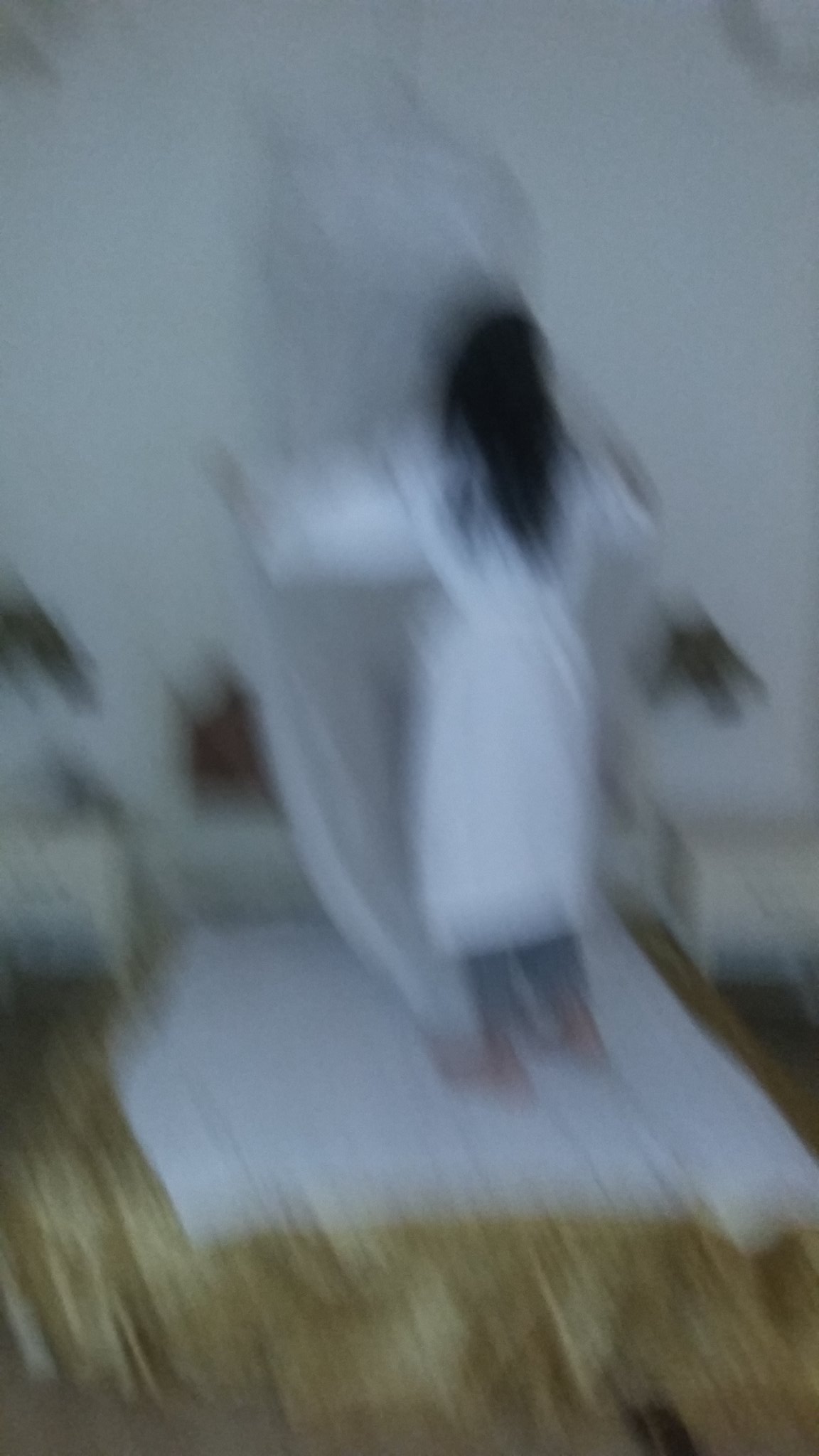In this very blurry color photograph, a woman with long black hair, wearing a white robe and gray leggings, stands barefoot on a white rug that covers a shiny, light brown hardwood floor. She faces an off-white wall with her back towards the viewer, her hair reaching halfway down her back. One hand is raised to her side while the other hangs down. The scene appears to be indoors, likely in a bedroom, with hints of bedside furniture obscured by the poor focus. The photo is vertical, rectangular, and low resolution, giving an impression of motion or activity by the woman.